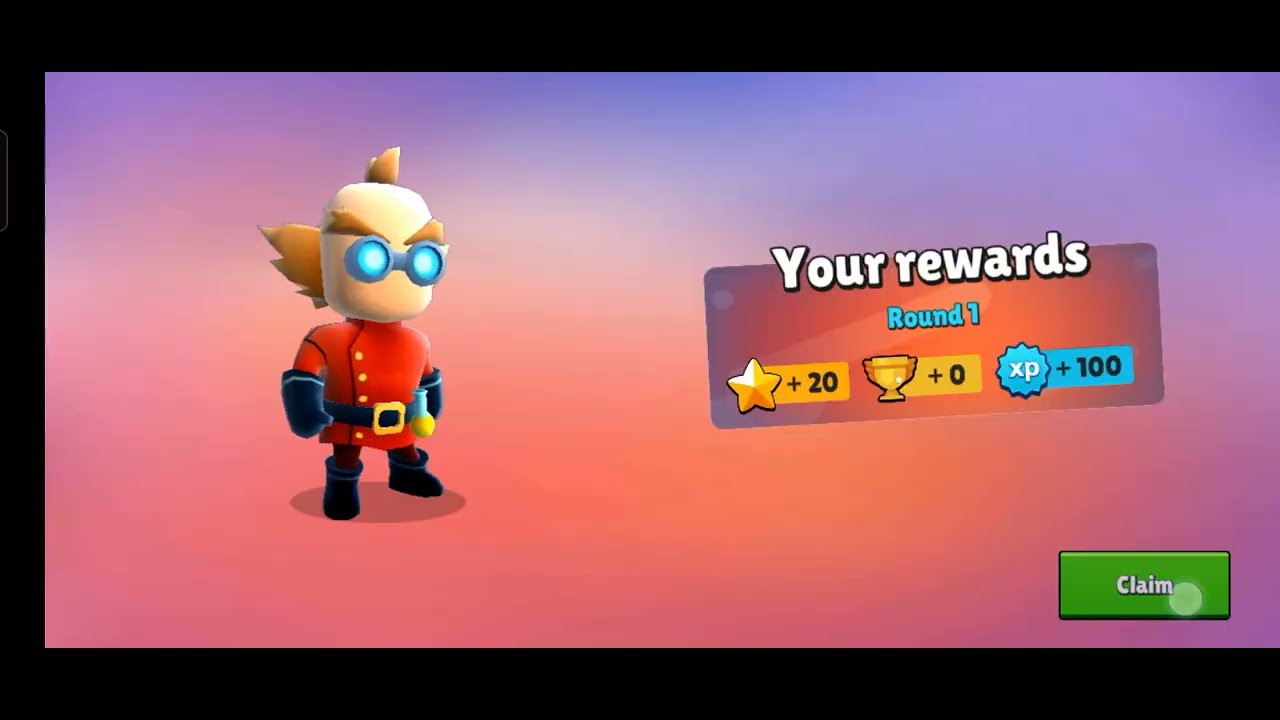The image appears to be a screenshot from a video game, showcasing a vibrant, colorful reward screen. The background features a gradient transitioning from purple at the top to a mix of orange and purple towards the bottom. Along the border runs a thick black line that frames the content.

In the left-center of the image stands a steampunk-styled cartoon character resembling an old military redcoat. He is wearing a distinctive Park Ranger-like outfit with a deep red jacket adorned with gold buttons, a black belt with a gold buckle, and clunky black boots. The character also sports silver rounded goggles, a brown mohawk with side hair, big black gloves, and carries a yellow flask.

To the right-center of the screen, a prominent box labeled "Your Rewards" in white text displays the game's round one rewards: a star icon with "+20," a trophy icon with "+0," and an XP icon with "+100." Each item is vividly colored, predominantly in shades of blue and purple, with the text beneath them. At the bottom right corner of the image lies a green "Claim" button, inviting the player to collect their rewards.